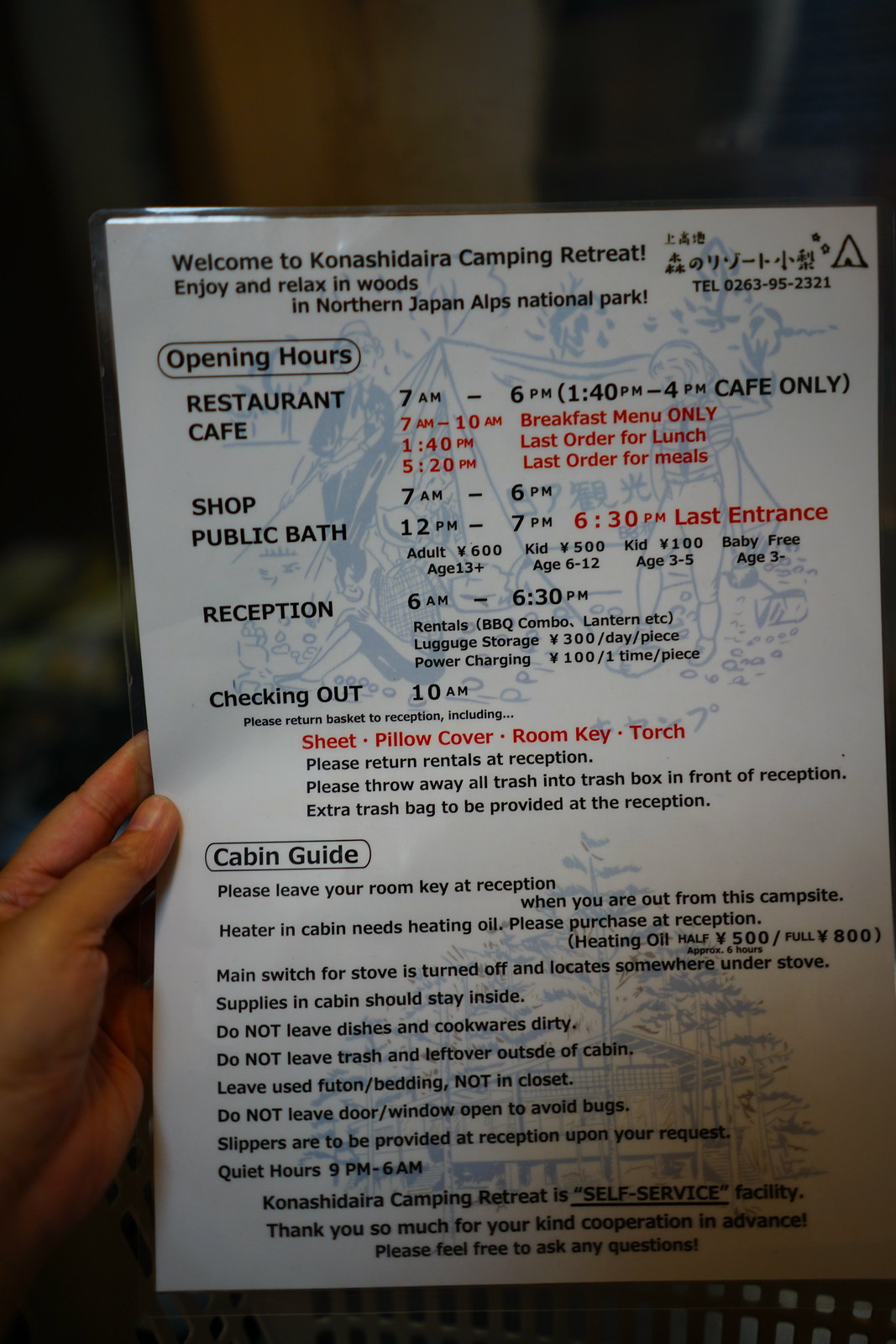The image shows a close-up photograph of a hand holding a laminated piece of paper. The hand, clearly visible on the left side, belongs to the person holding the paper. At the top of the document, in bold black text, it states, "Welcome to Konashidaira Camping Retreat." Below this, it reads, "Enjoy and relax in the woods in Northern Japan Alps National Park." The paper provides detailed information about the retreat's various amenities and schedules.

Underneath the welcome message, there is a section outlining the opening hours within a small circle bubble. It states "Opening hours" and provides the schedule for the restaurant cafe: 7 a.m. to 6 p.m., with a notation that from 1:40 p.m. to 4 p.m., it is cafe only. The cafe's specific hours are detailed: breakfast menu is available from 7 a.m. to 10 a.m., with the last order for lunch at 1:40 p.m., and the last order for meals at 5:20 p.m. The shop hours are listed as 7 a.m. to 6 p.m.

The document further includes information about additional facilities:
- Public Bath: 12 p.m. to 7 p.m., with the last entrance allowed at 6:30 p.m.
- Reception: 6 a.m. to 6:30 p.m., with check-out time at 10 a.m.

Following this, there is a Cabin Guide outlining the necessity to leave room keys at reception when leaving the campsite. It specifies that cabin heaters require heating oil, which can be purchased at the reception, and mentions the location of the main switch for the stove. The guide also reminds guests to keep all supplies inside the cabins and not to leave dishes or trash outside as it is a self-service facility.

Additionally, in the top right corner of the paper, there is some Chinese writing and below it, a telephone number: 0263-95-2321. The bottom of the form thanks guests for their cooperation and invites them to ask any questions they might have.

Overall, the laminated paper provides comprehensive details about operating hours, amenities, and guest responsibilities, ensuring a comfortable stay at the Konashidaira Camping Retreat.